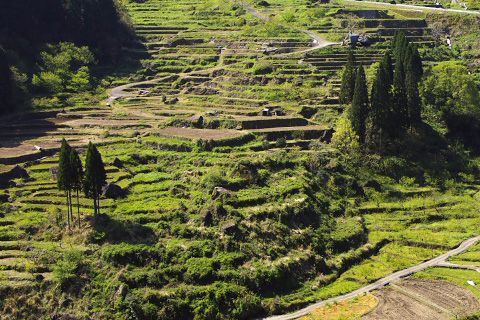This image captures an aerial view of a picturesque, tiered countryside landscape, reminiscent of an Italian orchard. The hill dominates the scene, gradually descending with distinct, stone-like layers that create a staircase effect. Each tier is densely blanketed with lush green grass. In the midsection of the hill, the stone slabs are visible, adding texture to the verdant expanse. To the right side of the image, a cluster of tall, cypress-like trees stands prominently, while the left side features fuller green trees. A notable dirt patch is observable in the lower right quadrant, where a network of grey roads traverses the landscape, connecting various parts of this idyllic agricultural setting.